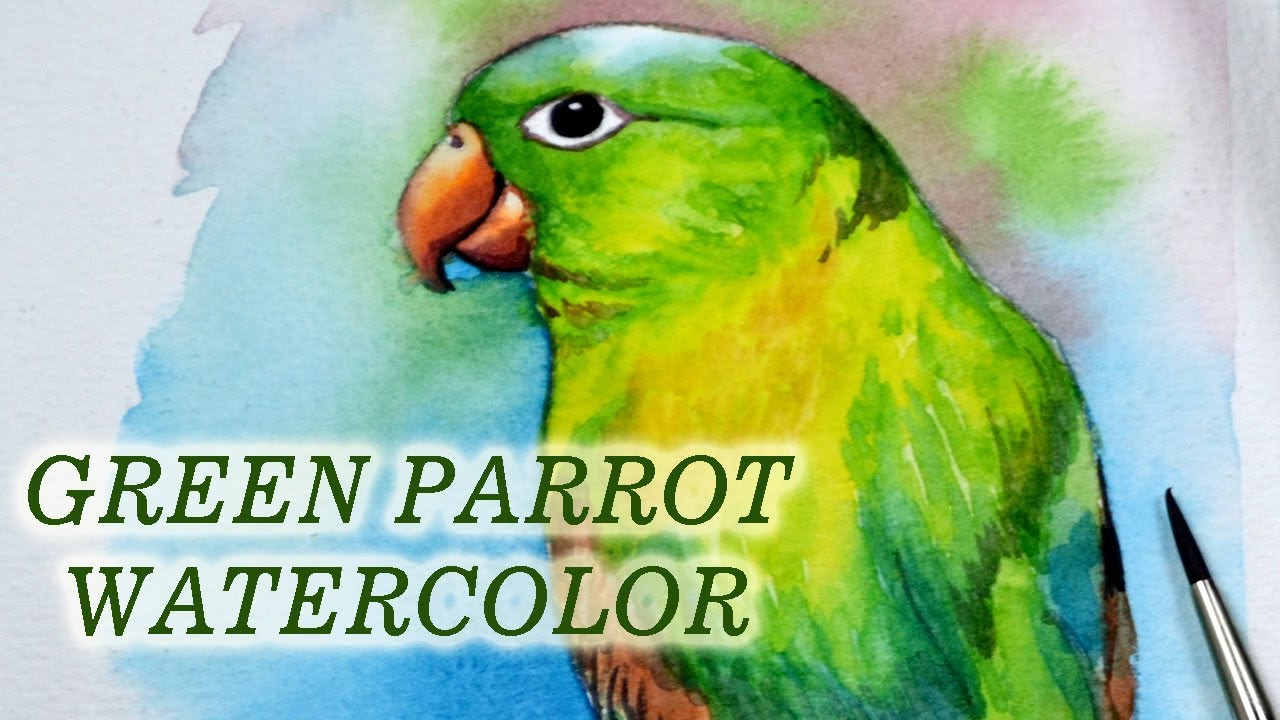The image features a vibrant watercolor illustration of a green parrot, prominently positioned in the center right, facing to the left. The parrot is adorned with an array of hues; its head is light green, grading to yellow around the neck, while the wings showcase a spectrum of light green, blue, and subtle brown, with red and yellow accents. The parrot’s beak is orange, and its left eye, which is white with a black pupil, gazes directly at the viewer. The belly and underside of the bird display shades of light brown and orange. The background is a fluid mix of watercolor stains in blue, pink, green, and red tones, fading out to white at the edges, all on textured watercolor paper.

A green serif font with a soft white glow text in all capital letters reads "GREEN PARROT WATERCOLOR" on the bottom left corner of the image. A watercolor paintbrush rests beside the parrot in the bottom right corner, adding an artistic touch to the scene.